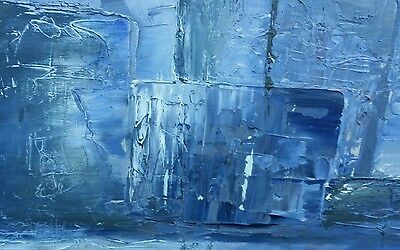The image is a watercolor painting predominantly showcasing a range of blue hues, varying from light blues to dark blues, and interspersed with patches of white and hints of gray. The composition features three ice cubes, with the cube in the center slightly smaller than those on either side. The ice cubes appear to be reflecting light, creating a shiny effect that adds to their icy look. The lower right-hand corner of the painting introduces a moldy green backdrop behind a lighter blue area, forming a distinct rectangular shape. The entire scene is set against a ground of similar colors, giving an impression that the ice cubes are possibly melting, as if situated in a puddle of water. Abstract in nature, the painting includes numerous small white scratch marks adding texture to the overall design. While lacking an artist's signature, this modern piece skillfully uses varying shades and reflections to evoke a chilling, lifelike representation of melting ice cubes in a modern abstract style.